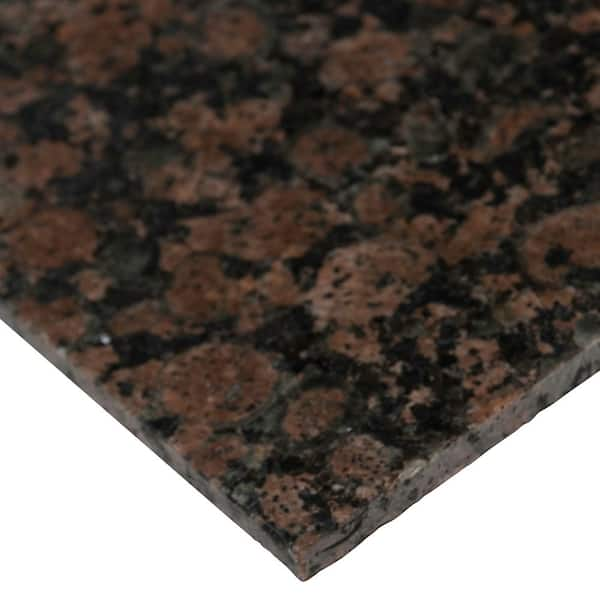This image features a close-up of a granite countertop corner presented against a white background. The countertop forms an upside-down pyramid shape with the granite extending upward and filling the rest of the photo. The stone surface exhibits a detailed, marble-like pattern composed of a mix of browns and blacks, interspersed with hints of reddish hues that contribute to its intricate, grizzled texture. The countertop resembles the shape of a home run base from baseball, with its edge clearly defined and dipping toward the bottom of the screen in a V shape, highlighting the textured surface.